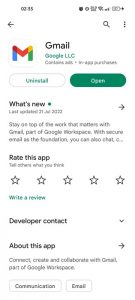The image depicts the Google Play Store interface on a smartphone, showcasing the Gmail app. The Gmail icon is positioned at the top left of the screen with a white background and features a multicolored 'M' in blue, red, yellow, and green. Adjacent to the icon, "Gmail" is written in black. Just below, in green text, it reads "Google LLC," followed by black text indicating that the app contains ads and offers in-app purchases.

Further down the screen, there are two buttons. The left button, with a white background and green text, reads "Uninstall," while the right button has a green background with white text that reads "Open." Beneath these buttons, a section titled "What's New" is displayed, stating that the app was last updated on 21 July 2022 and mentioning the new features: "Stay on top of the work when part of Google Workspace with secure email SD."

Continuing down, there is a segment encouraging users to "rate app" with five stars, which are currently grey, indicating they are not rated. "Write a review" is prominently in green below the stars. At the very bottom of the image, black text details further sections: "Developer Contacts" and "About This App," which describes Gmail as part of Google Workspace and highlights its capabilities to connect, create, and collaborate. Lastly, two categories, "Communication" and "Email," are visible at the bottom, both with white backgrounds.